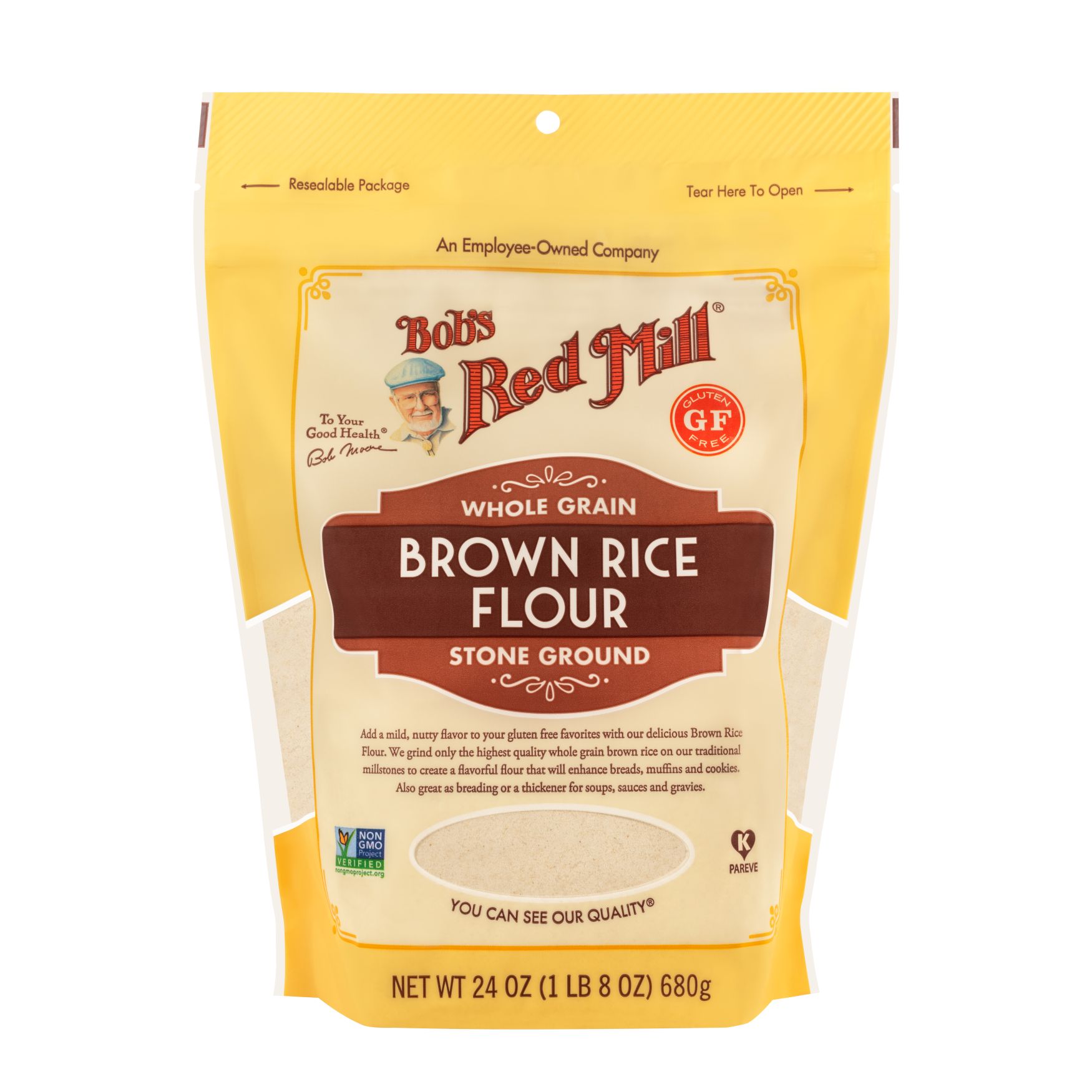The vividly detailed image showcases a vertically oriented package of Bob's Red Mill Whole Grain Brown Rice Flour. Dominated by a gold background, the package features a central cream-colored rectangular panel accented by prominent red and brown text. At the top, the red script reads "Bob's Red Mill," accompanied by a charming illustration of Bob himself, donning a blue cap and gray beard, with the phrase "To Your Good Health" and his signature beside it. The package is notably gluten-free, as indicated by the "GF" label beneath the brand name. Below this is a series of labels in shades of brown: "Whole Grain" in white text on a lighter brown shield, "Brown Rice Flour," and "Stone Ground" in dark brown strips. A descriptive blurb emphasizes the flour's mild, nutty flavor and its suitability for gluten-free baking and cooking. Unique to the design is an elliptical transparent window near the bottom, giving a clear view of the flour inside, with the reassuring text, "You Can See Our Quality." Finally, the net weight of 24 ounces (1 pound, 8 ounces, or 680 grams) is clearly marked at the package's base. The product, contained within a resealable, tear-open bag, underscores the brand’s commitment to quality by noting its employee-owned status at the top. This meticulous real-world package design is a testament to the brand's dedication to transparency and health.